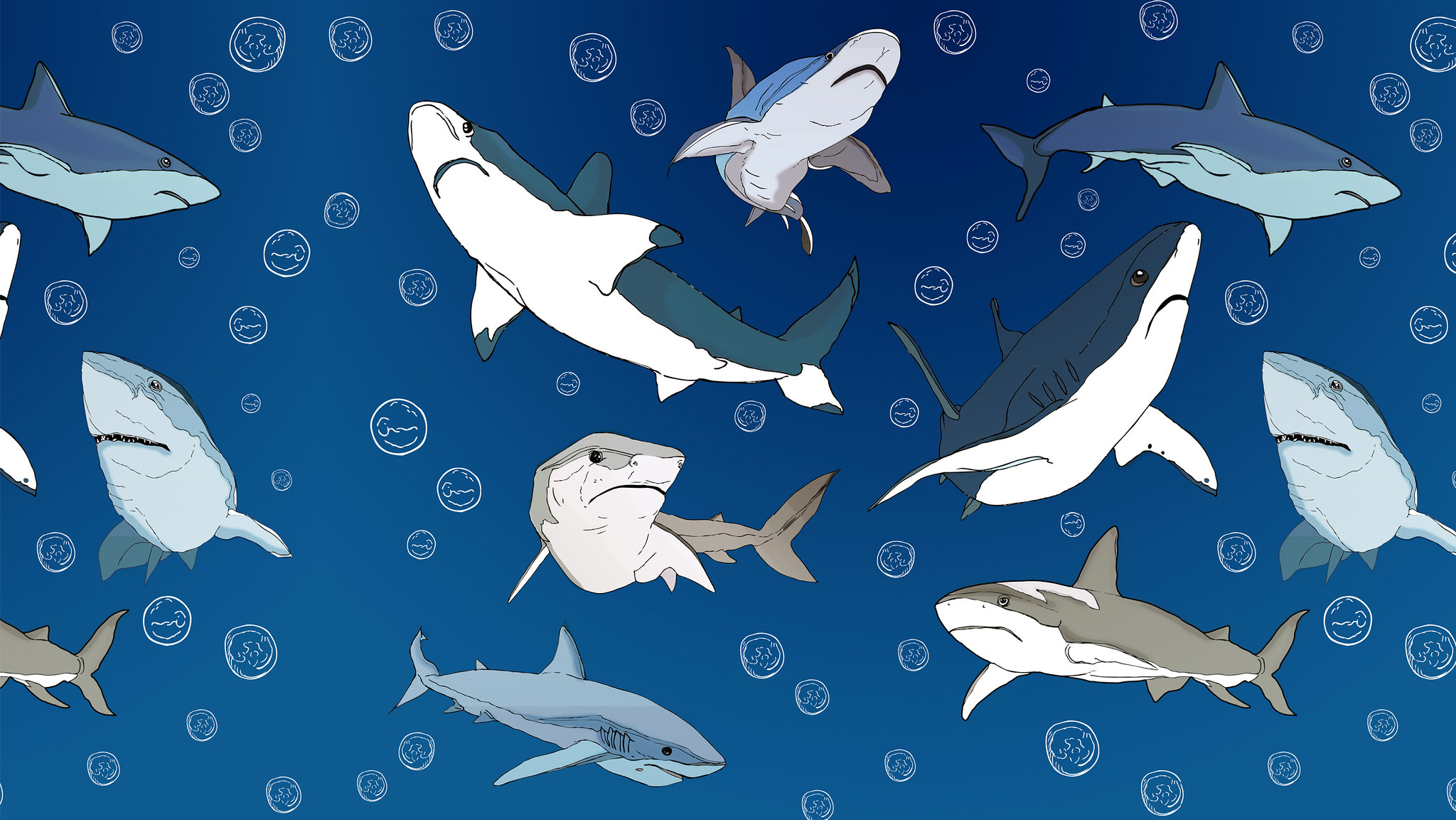This digital artwork depicts a captivating underwater scene featuring various species of sharks in a mid-swim. Scattered throughout the dark-to-light blue gradient background, the sharks are portrayed in different positions, showcasing a diverse array of species such as tiger sharks, whale sharks, and great white sharks, along with some unidentified types. The sharks' color palette ranges from gray and blue to turquoise, with many exhibiting white underbellies. Their mouths are mostly closed, adding a serene quality to the scene. The composition gives the impression of viewing a school of sharks from below, looking up towards the surface. Adding to the aquatic ambiance, numerous white bubbles are dispersed throughout the image, enhancing the sense of depth and movement in this underwater tableau.